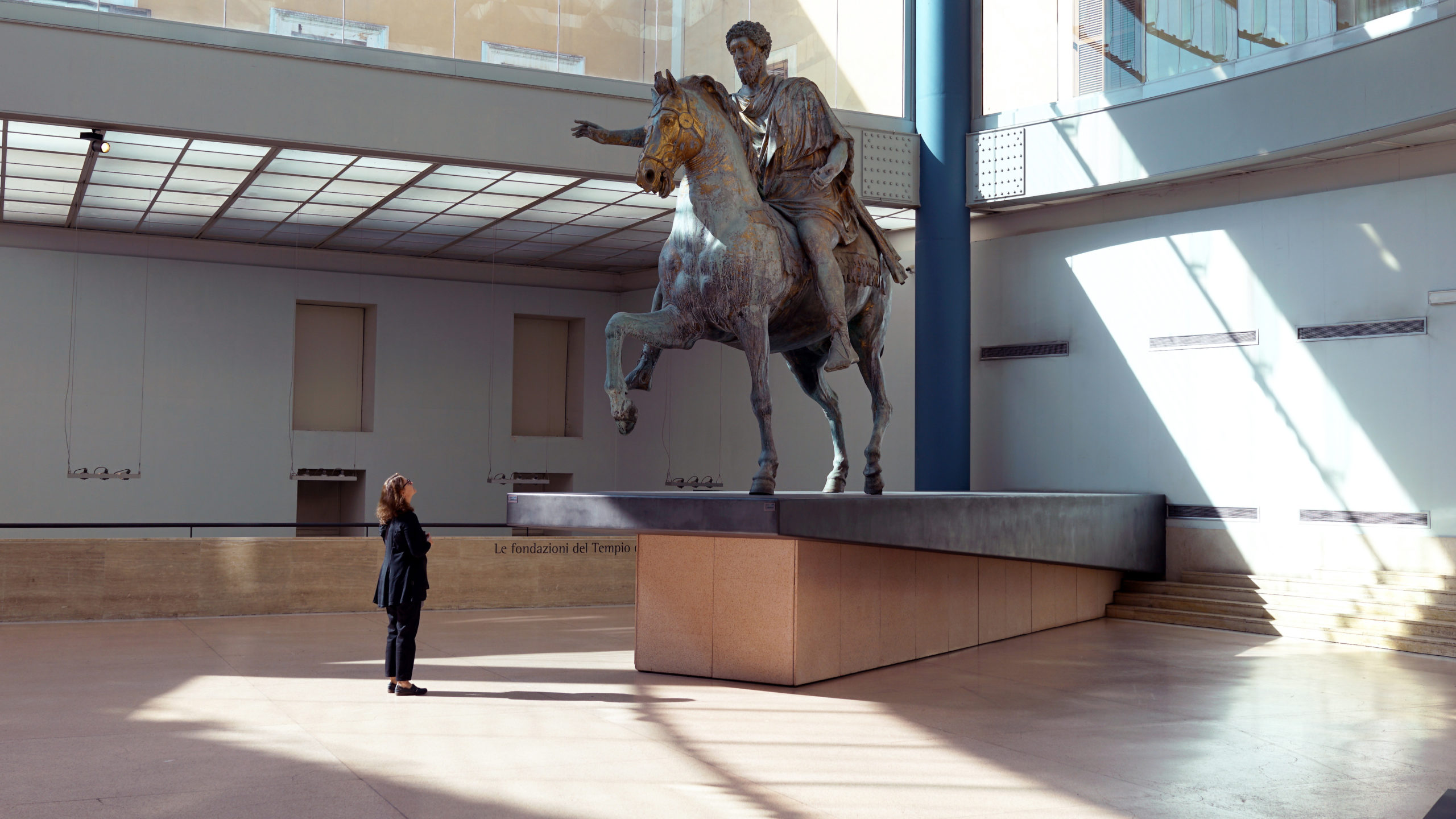In this photograph, a woman stands in a museum with cream-colored, slightly reddish concrete floors and gray walls, illuminated by natural light streaming through large upper-floor windows. She is the sole figure in the image. The woman, a white lady with shoulder-length brown hair and glasses, dons a black jacket, navy pants, and black shoes. She gazes upwards at an impressive bronze statue on a long platform before her. The statue depicts a man with curly hair and a beard, draped in a Roman-style tunic and sandals, riding a horse with its right front leg raised. A blue column stands prominently in the background, and some visible text reads "La Fendoceno del Tempio," suggesting the museum might be located in a Spanish-speaking country. The spacious room is well-lit, with light filtering through ceiling-high glass windows.